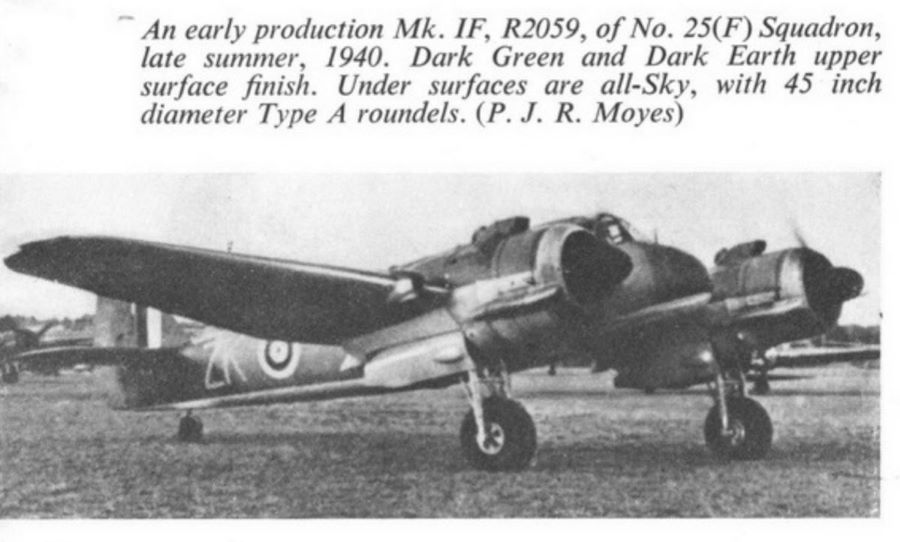This image features a color photograph of a black and white image from a newspaper or magazine. The top half consists of black text on a white background, providing detailed information about the aircraft depicted below. The lower half showcases a grainy black and white photograph of an early production MKIF R2059 of Number 25F Squadron from late summer 1940. The airplane appears to be an old propeller plane likely from the 1940s, though it might even date back to the 1930s. The aircraft, which appears small and possibly designed for one or two people, has distinctive markings, including "ZK" painted on the side. It features a two-wheel setup at the front and a single wheel at the back. The text specifies the aircraft's color scheme with a dark green and dark earth upper surface finish, and "sky" colored undersurfaces adorned with 45-inch diameter type A roundels. The text is credited to PJR Moyes. This historical plane likely saw action during World War II, reflecting its era through its design and detailing.